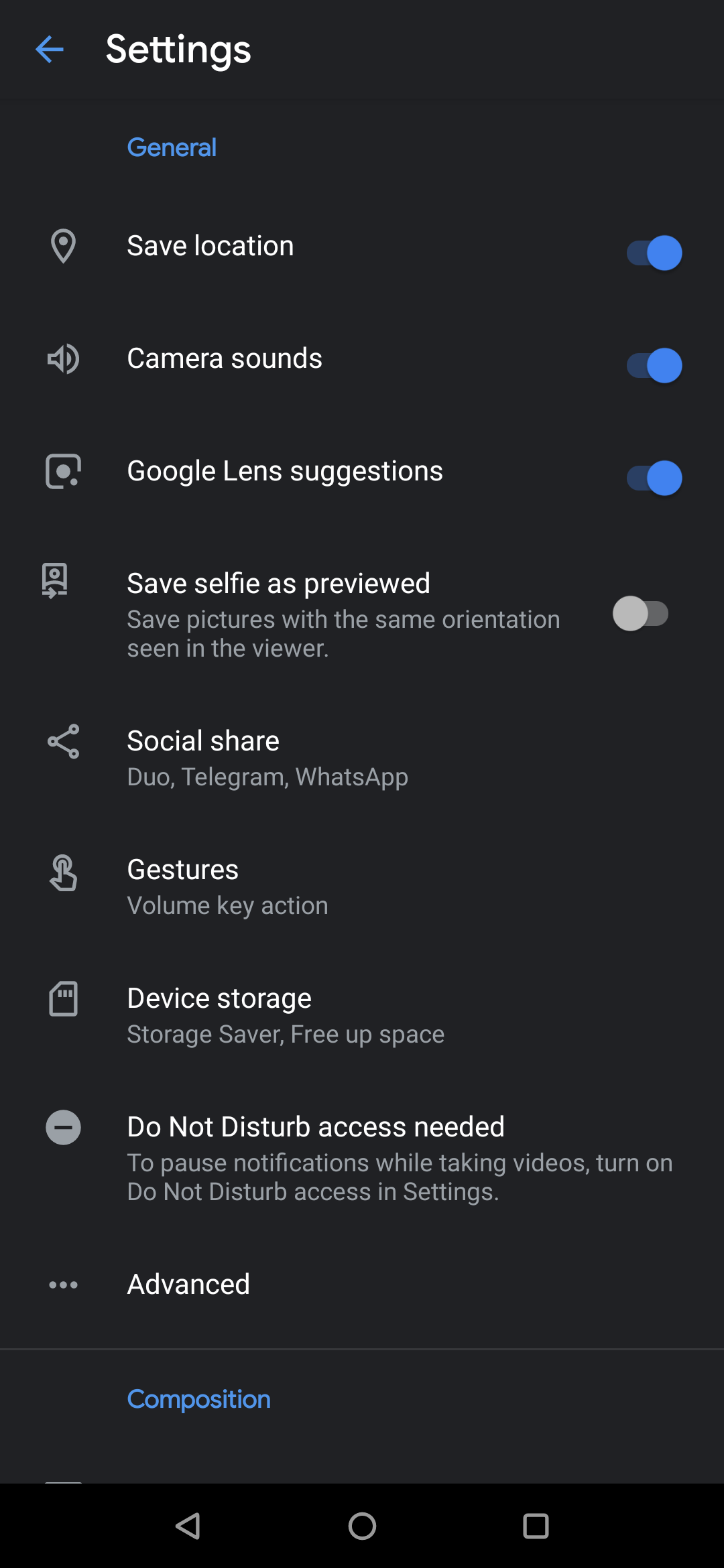**Detailed Caption:**

The image captures a screenshot of a settings page on a mobile device. At the very top of the screen, there is a section with a dark gray background. In the center of this section, the word "Settings" is prominently displayed in white text. On the left-hand side of this top bar, a blue left-facing arrow symbolizes a 'back' function.

Below the "Settings" title, a smaller blue font reads "General." A list of settings follows, each item displayed in white text:

1. **Save Location**
2. **Camera Sound**
3. **Google Lens Suggestions**
4. **Save Selfie as Previewed** - accompanied by the description "Save pictures with the same orientation seen in the viewer."
5. **Social Share** - with options listed as "Duo, Telegram, WhatsApp."
6. **Gestures** - described as "Volume key action."
7. **Device Storage** - includes "Storage saver, free up space."
8. **Do Not Disturb Access Needed** - with the note "To pause notifications while taking videos, turn on Do Not Disturb access in settings."

To the right of the first four settings (Save Location, Camera Sound, Google Lens Suggestions, and Save Selfie as Previewed), there are toggle buttons. These buttons can be slid to the left (off, shown in gray) or to the right (on, shown in blue). In the screenshot, Save Location, Camera Sound, and Google Lens Suggestions are toggled on (blue), while Save Selfie as Previewed is also toggled on (gray).

Each setting is accompanied by an icon on the left, signifying its function. For example, location and camera sounds have their respective logos.

Under the "Do Not Disturb Access Needed" setting, the word "Advanced" appears in white letters, accompanied by three horizontally aligned gray dots signifying a menu or additional options. Beneath this section, a very thin gray line marks a separation.

Further down, the word "Composition" is displayed in blue text, followed by the bottom border of a typical mobile device interface. This border is black and rectangular, containing three icons: a back button (a left-pointing triangle), a home button (a circle), and a square button for recent apps, all outlined in gray.

This descriptive caption provides a thorough representation of the settings page, highlighting the interface elements and their respective details.